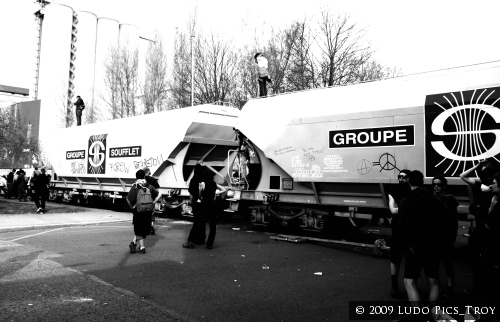A black and white photograph captures an outdoor scene with a long train prominently featuring graffiti and logos. The train appears to consist of multiple white carts, each adorned with logos including "GROUPE" in white text on a black rectangular background, and another square logo with the letter "S" and vertical lines. A third logo, reading "SOUFFLE," is also present in white text on a black rectangular background. The train has peace symbols and other graffiti, including an anarchy-inspired "A=peace" symbol. 

The scene includes various men and women on and around the train. Some individuals stand atop the train carts, creating a juxtaposition with the people walking and gathering on the asphalt below. People on the ground include a mix of those with and without backpacks. The surroundings suggest an open area with vertical elements that might be street lamps or pillars, complemented by a backdrop of trees and possibly buildings, though the monochromatic nature of the image obscures finer details. Shadows cast on the asphalt add depth to the composition. The bottom right corner of the photograph bears a watermark reading "© 2009 Ludopix Troy," indicating the image's origin. The overall mood, combined with the presence of watchful individuals, evokes a sense akin to a surveillance or Big Brother atmosphere.